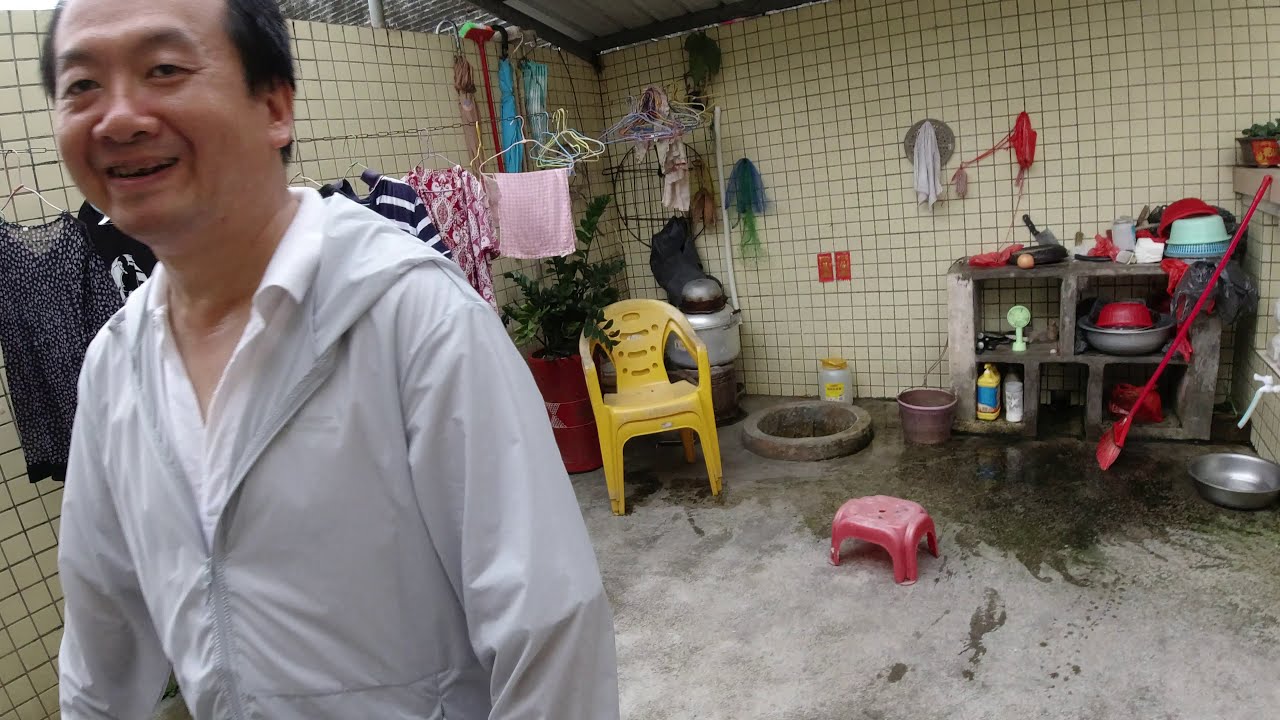The photograph depicts a middle-aged Asian man dressed in a gray hoodie over a white V-neck shirt, standing in the foreground on the left side of the image. He is smiling warmly at the camera. The setting appears to be an indoor work area or kitchen with distinctive white or light yellow tiles covering the walls. Behind him, there is a rack holding various clothing items, partially obscured by his shoulders. Adjacent to this, two stackable yellow resin chairs are placed on the floor. In front of these chairs, there is a cement floor that has become wet.

To the right of the man, the scene includes a clutter of cleaning utensils and tools. These include hanging towels, a red broom or mop leaning against the wall, and a silver cleaning container. A small red step stool is positioned centrally on the floor with a tire of a work cart, a brown bucket, and an open cabinet containing liquid cleaning supplies nearby. Further to the right, there is a cement work table built with shelf-like openings, hosting various kitchen items, including stacked silver and red bowls. A hole in the floor is visible next to the bucket. The space feels utilitarian with a mixture of stored items and cleaning equipment, suggesting it's a multi-functional area possibly connected to a house or workshop.